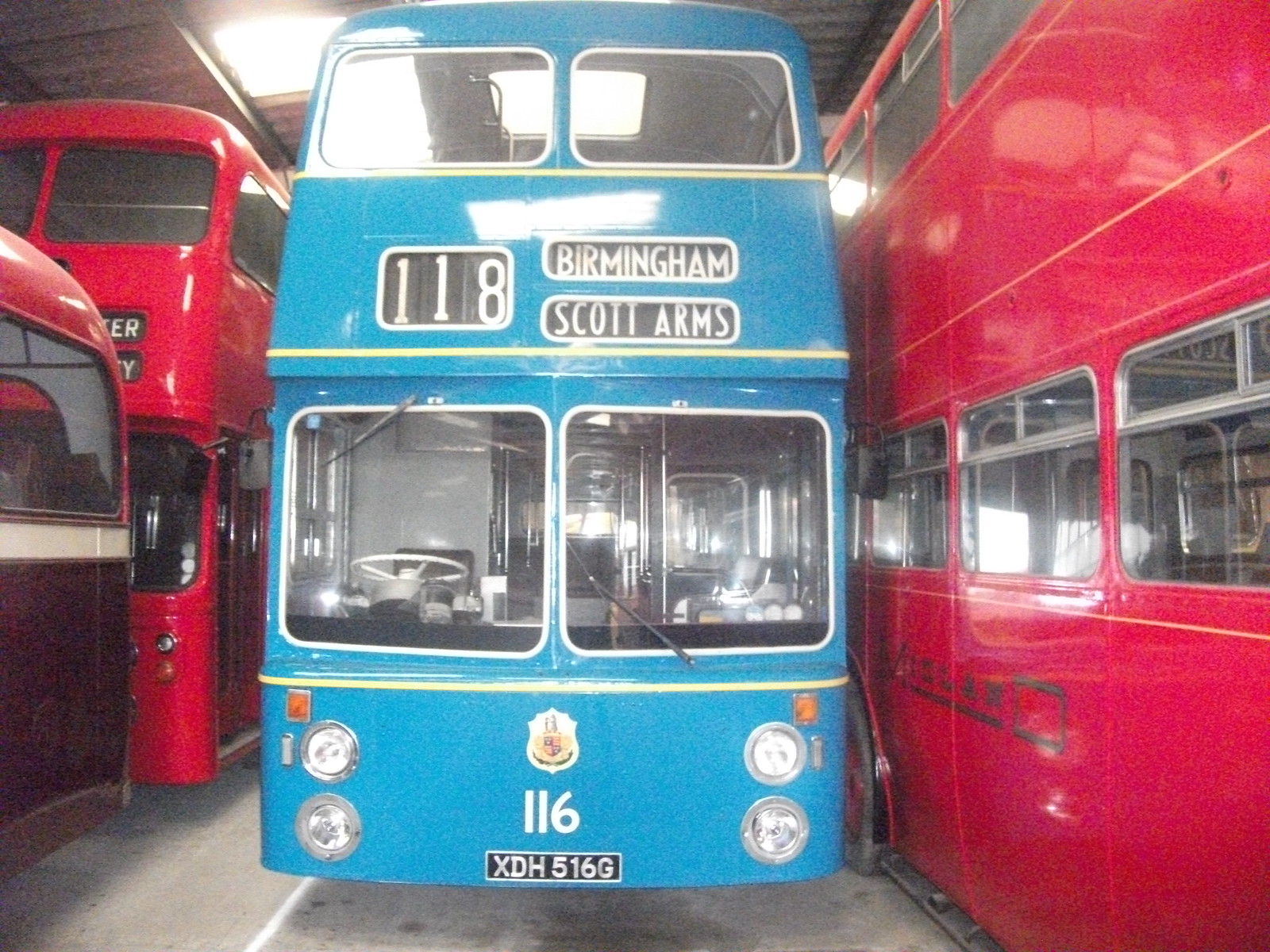The image is a full-color photograph taken inside a large parking garage or warehouse designed for vehicles. The floor is light gray concrete, and above is a corrugated metal roof equipped with fluorescent lighting that provides a stark illumination. Dominating the center of the frame is a bright blue double-decker bus, prominently displaying the number "118 Birmingham Scott Arms" in white text on a black background at the front. Beneath this, a coat of arms and the number "116" are also visible. The blue bus bears a European-style license plate marked "XDH-516G" in black with white lettering. The windshield is split into two square segments, and four distinct headlights can be seen below it. 

Flanking the blue bus on both sides are large red double-decker buses, invoking the classic image of London transport. To the left of the blue bus, part of a smaller vehicle, possibly another bus, is partially visible. All the buses appear empty, and their polished exteriors capture the industrial ambiance of the garage. The entire setting, accentuated by the reflections and the orderly arrangement of the buses, suggests a well-maintained and organized storage area.